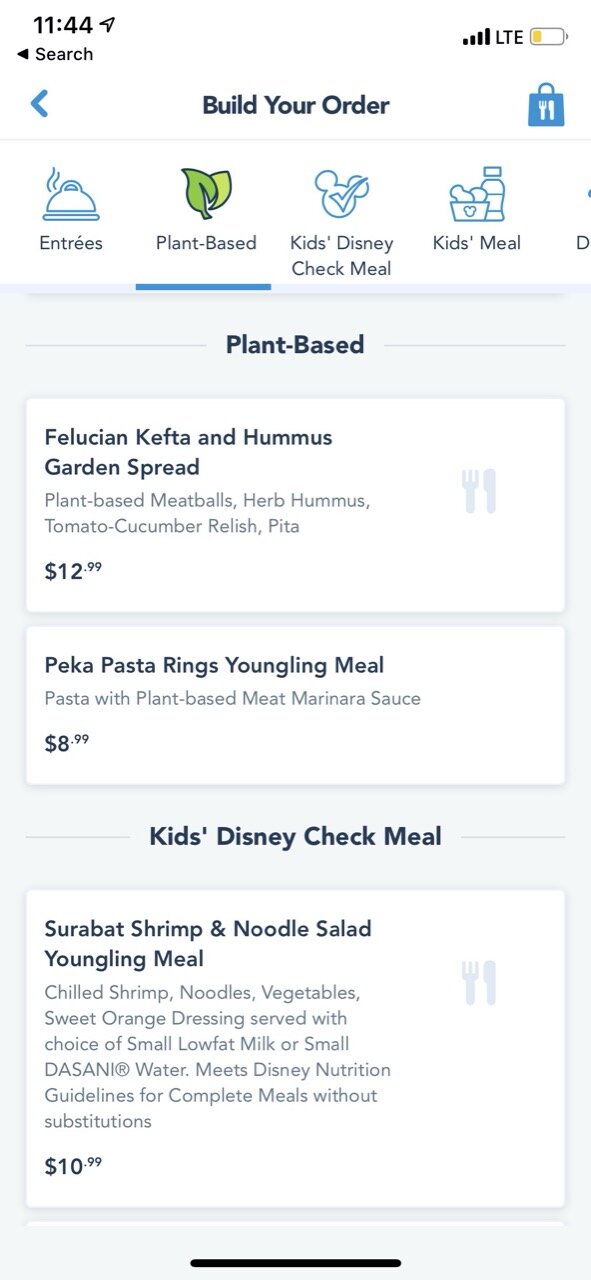Here's a cleaned-up and detailed caption for the image:

---

The image displays a smartphone screen running a food ordering app. The top portion of the screen has a white background, transitioning to a very pale blue background covering the bottom two-thirds of the screen. 

At the upper left corner, the time is displayed as "11:44" with a search icon and a left arrow just below it. On the top right, the signal strength shows four out of four bars, labeled "LTE," next to a battery icon with a yellow bar indicating a low battery level.

Just beneath this top bar is a thin line, with a bold left-pointing arrow situated on the left side. On the right side, there is a blue shopping bag icon featuring a fork and knife, identifying this as a food ordering app.

Centered on the screen in bold black letters is the title "Build Your Order," followed by a faint gray line stretching across the screen. Below this, a row of icons represents different food categories: "Entrees," "Plant-based," "Kids Disney Check Meal," "Kids Meal," and an option partially cut off starting with "D."

- The "Entrees" icon is a blue outline of a covered dish with steam rising.
- The selected "Plant-based" option has a full-color icon showing a light and dark green leaf, indicated by a blue underline.
- The "Kids Disney Check Meal" features a blue outline of a Mickey Mouse head with a check mark.
- The "Kids Meal" icon appears as a blue outline of a juice bottle and a bowl with nuggets.

The "Plant-based" section is active, occupying the pale blue background. It starts with a black title "Plant-based" and contains three white text rectangles, each with dark blue text:

1. **"Felucian Kefta and Hummus Garden Spread"**  
   Plant-based meatballs, herb hummus, tomato cucumber relish, pita  
   **Price: $12.99**  
   Accompanied by a pale blue fork and knife icon on the right.

2. **"Peka Pasta Rings Youngling Meal"**  
   Pasta with plant-based meat marinara sauce  
   **Price: $8.99**

3. **"Surabot Shrimp and Noodle Salad Youngling Meal"**  
   Chilled shrimp, noodles, vegetables, sweet orange dressing, choice of small low-fat milk or small Dasani water, meets Disney nutrition guidelines for complete meals without substitutions  
   **Price: $10.99**  
   Accompanied by a pale blue fork and knife icon on the right.

The bottom portion of the screen features a black bar running across the middle third.

---